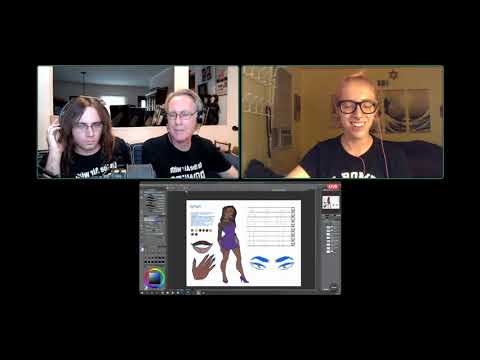The image features a Zoom call screenshot divided into three panels, with the top half consisting of two side-by-side panels and the bottom half displaying a single panel. In the top-left panel, two individuals are engaged in conversation, both wearing black t-shirts with white lettering and headphones. The woman on the left has long brown hair, glasses, and a center part, while the man on the right has short gray hair, glasses, and a faint view of a room behind him. The top-right panel spotlights a smiling blonde woman with her hair up in a ponytail, wearing thick-framed black glasses and a black t-shirt with white text. Her eyes are closed, and she appears to be looking at the screen. The bottom panel shows a computer screen with an open image editing software displaying a woman in a purple dress and various disembodied body parts, including a hand, lips, and eyes with blue eyebrows.